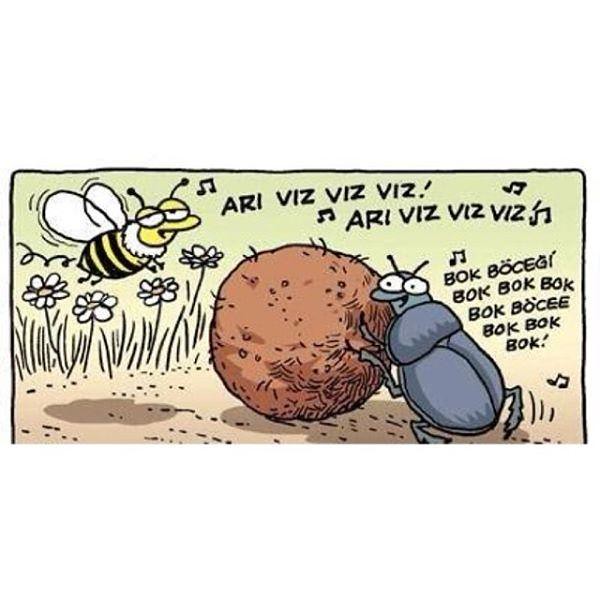The cartoon illustration features a vibrant scene with a dung beetle and a bee. On the right side of the image, a bluish-gray dung beetle with large, expressive eyes is energetically rolling a small brown ball of dung, seemingly singing with lyrics that read "Bok, bok, bok, bok, bok, bok, bok, bok" accompanied by musical notes. To the left, a sleepy-looking bee with droopy eyelids, adorned in black and yellow stripes, hovers above some short dark strokes symbolizing grass and white-leaved dandelions. The bee is also singing, with the text "Ari, viz, viz, viz, Ari, viz, viz, viz" and more musical notes floating around. The ground beneath them is depicted in brown with a few shadows that accentuate their positions, creating a whimsical and lively scene.